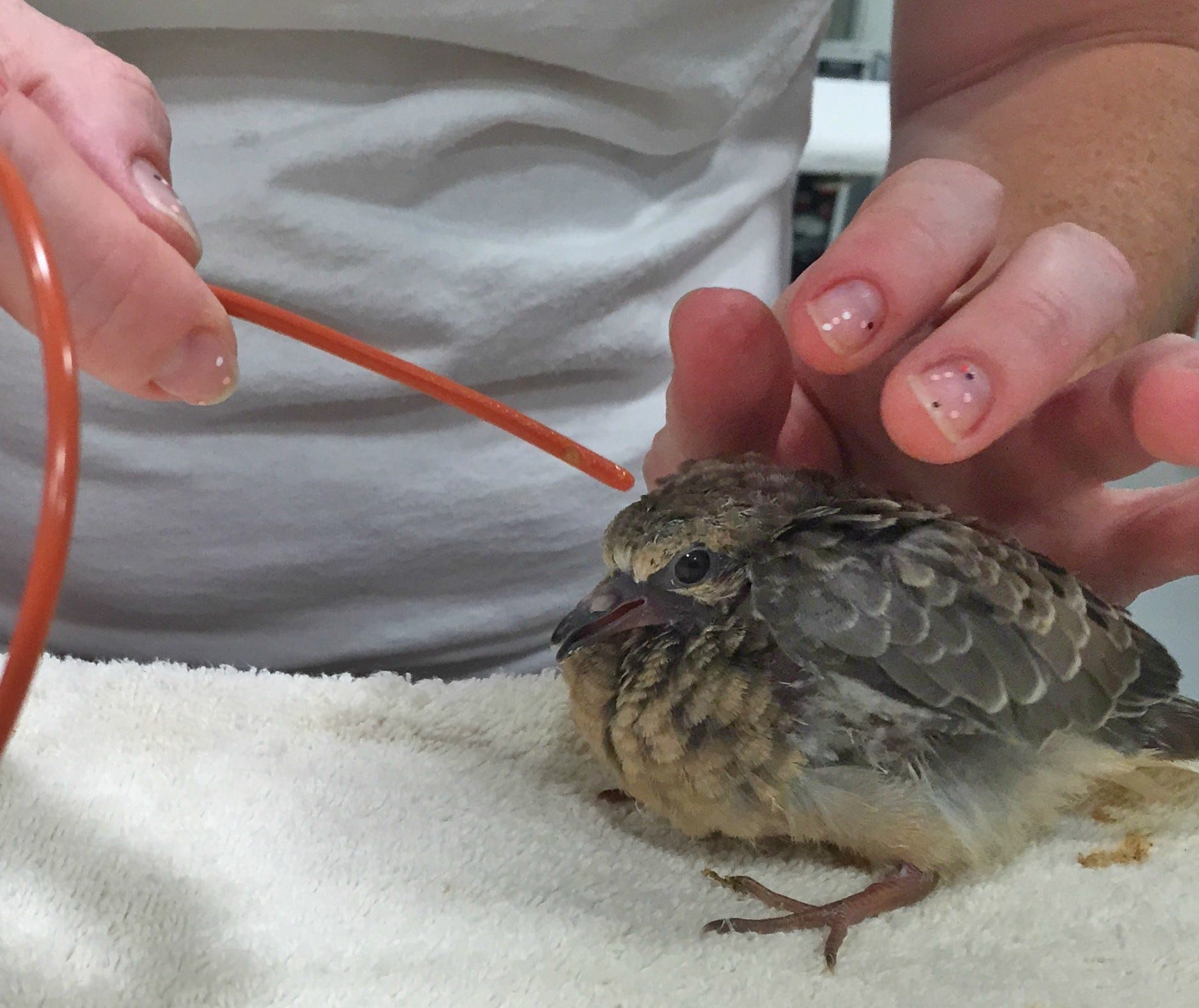The image captures a small, grayish-brown baby bird with a fluffy tan-gold breast, sitting calmly on a white terry cloth towel. The bird appears to be in a care setting, possibly a veterinarian office or a nature center, and has its legs splayed out slightly, giving it a puffed appearance. Its feathers are ruffled, making it look very cute and endearing. 

In the foreground, a person—likely a veterinarian or an assistant—wears a white t-shirt. Only their hands and the lower part of their shirt are visible. The individual's hands, adorned with glittery nail polish and small black flecks, gingerly approach the bird. They hold a dull orange plastic tube, which they are directing towards the bird, perhaps to administer a treatment or feed it. The scene is delicate and patient, and the bird shows no signs of distress, indicating a careful and compassionate interaction.